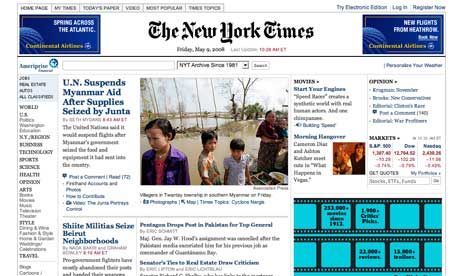This is an image of the New York Times website, primarily square or slightly horizontally rectangular in shape. The general background is predominantly white. At the very top, there is a white section containing six buttons with a light gray background and black lettering. These buttons are aligned from the top left towards the middle. Difficult to read due to small and blurred text, the rightmost button seemingly says "Try Electronic Something," followed by "Log In" and "Register Now".

Below this section, two blue rectangular areas with logos are present on the left and right. The left one contains the text “Spanning Across the Atlantic” in white letters, while the right one reads “New Flights from Heathrow.” Between these two is a large, white rectangular space with "The New York Times" prominently displayed in black letters. In smaller, unreadable text, more information is positioned below this heading.

A thin black line separates this banner from the content below. On the left side, a vertical menu features clickable sections labeled with categories such as "World," "Health," "Sports," and "Technology."

Next to this, a larger square section contains an article. The headline reads, "UN Suspends Myanmar Aid After Supplies Seized by Junta." Accompanying the article is a large image depicting water, possibly from flooding or a river, with sparse trees and four individuals (two women and two children).

Further below, there are more articles, including one with the visible headline, "Shiite Militias Seize Beirut Neighborhoods," and another starting with “Pentagon Drops,” though the text is hard to decipher.

On the right side of the image, several areas are difficult to read, but there are sections related to "Markets" and a smaller picture featuring a couple of people. At the bottom right, there is a cartoonish representation of old film reels with black film strips and blue screens where images would be. However, the words within these sections are unreadable.